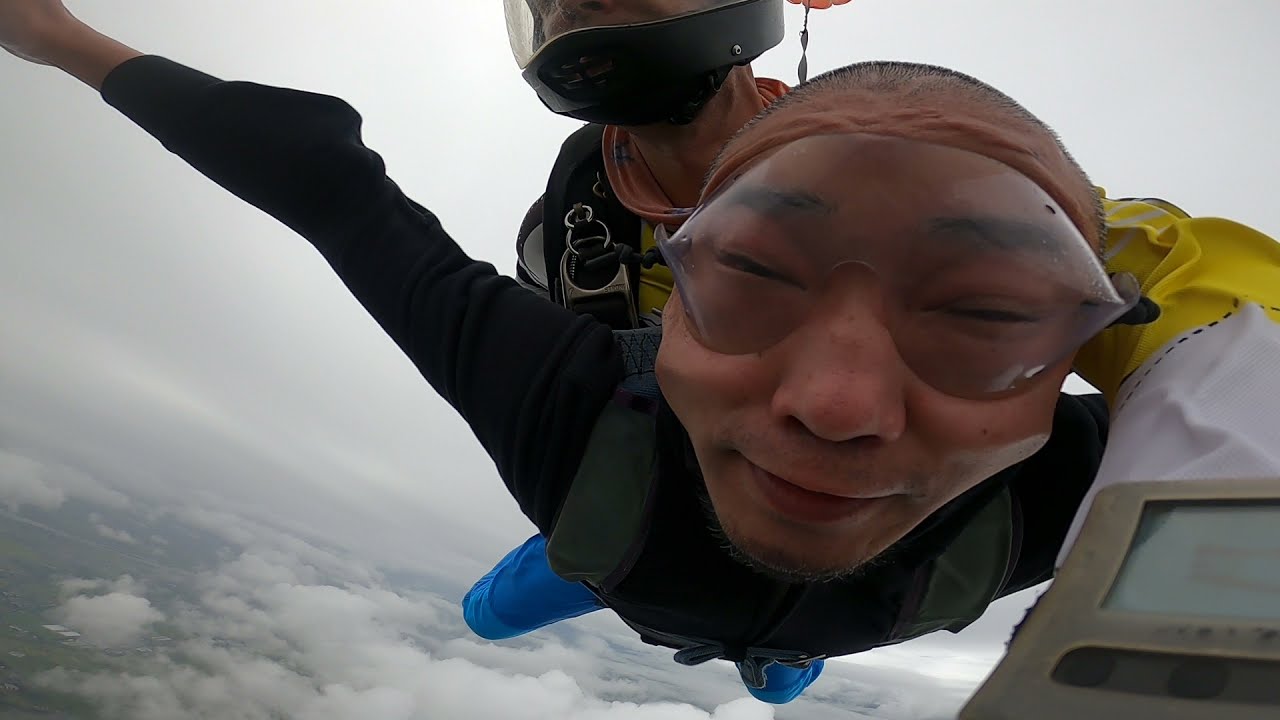The image captures the exhilarating moment of a tandem skydive from high above the Earth. At the center of the photograph is a man, possibly of Asian or Indian descent, with dark skin and a short buzz cut. He is smiling slightly, his face slightly distorted by the wind, and his dark eyebrows are visible above his clear goggles, which appear to have some moisture on them from either sweat or condensation. He has a small goatee and is wearing a black long-sleeve shirt. 

His arms are outstretched in a spread-eagle position, emphasizing the thrilling free-fall experience. Strapped to his back is a tandem instructor, only partially visible, identifiable by blue pants and a helmet. You can see part of the instructor's shoulder and leg, as well as an arm wrapped around the main subject's left shoulder, indicating the secure tandem harness.

The background features an overcast sky, with white clouds and patches of green land visible far below, particularly in the lower left corner of the image. The man, positioned to the right side of the frame, takes up most of the space and appears to be holding a camera to capture this unforgettable moment. Overall, the scene captures the excitement and intensity of the skydive, with the participant's joyful expression and the dramatic aerial backdrop.